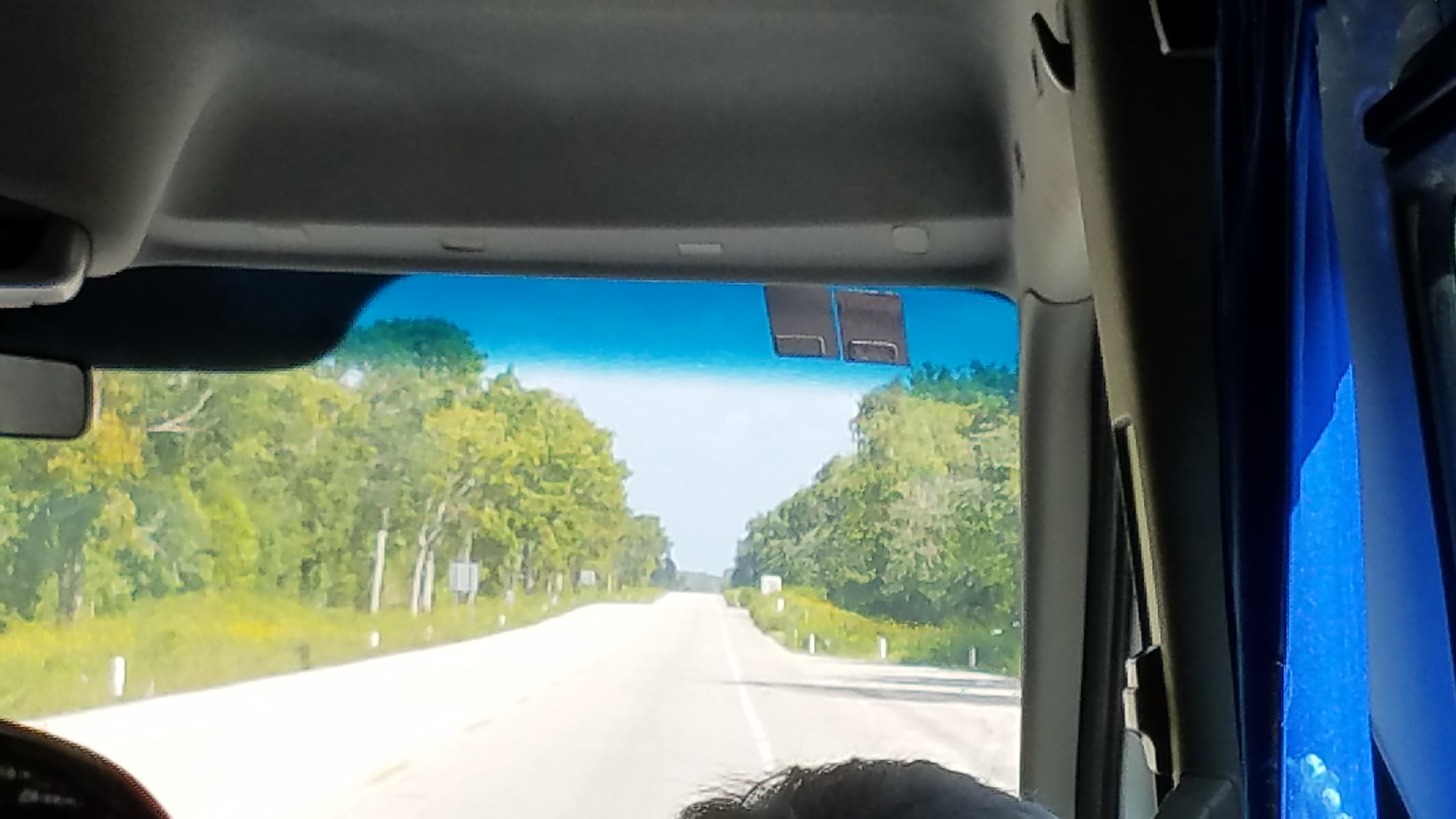This photograph, taken from inside a likely van or bus, captures the view through an off-centered windshield. The top portion of the windshield features a dark blue anti-reflective strip to minimize sun glare for the driver. Visible through the bottom edge of the image is the head of a passenger, seated on what appears to be the right side. Additionally, the seatbelt mechanism and a portion of the vehicle door are apparent, highlighting the spacious interior. The background reveals a bright, sunny day with a blue sky, lush green trees, and ample sunlight illuminating the road ahead.